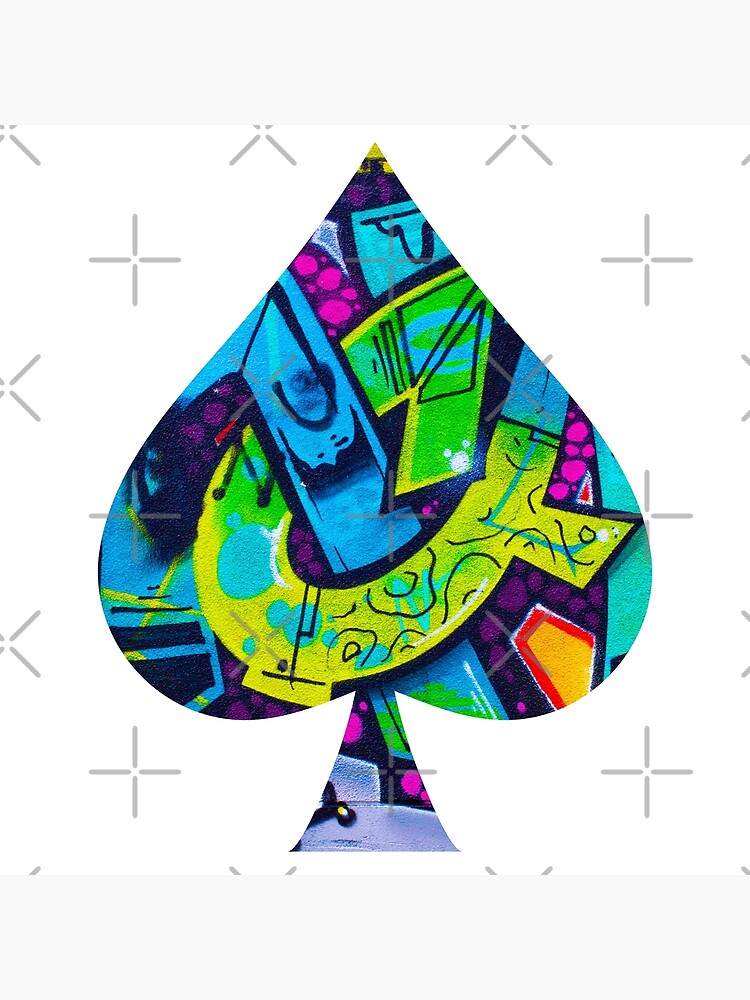This image features a striking painting of a spade symbol, prominently occupying the entire height and most of the width of the frame. Set against a black background scattered with repetitive gray X's, possibly as a deterrent to copywriting, the spade is vibrantly decorated with a polychrome abstract pattern evocative of 80s or early 90s graffiti art. The characteristic shape of the spade—which includes an upside-down heart merging into a pointed triangle—is intricately filled with a chaotic yet harmonious mix of colors including cyan, green, yellow, orange, purple, pink, and a darker blue, interspersed with patches of black.

Within this abstract mesh, certain patterns emerge, such as letter-like shapes that resemble interlocked L's and G's at the base, and an ambiguous Q in tones of yellow and lime green. Cyan lines morph into geometric forms like rectangles and trapezoids on the left, while an orange trapezoid with a red outline punctuates the right. Also notable are pink grape-like forms at the top left and a representation of an upside-down mountain within a cyan rectangle near the tip. The spade is capped with a yellow tip, adding to its vibrant complexity and making it a captivating piece of decorative clip art.